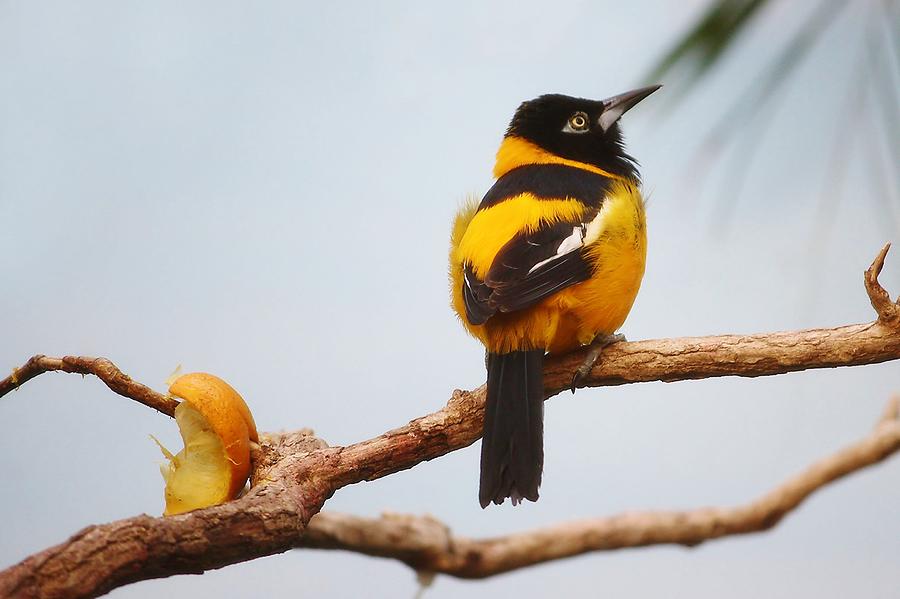In the image, a bird perches on a large tree branch extending across the entire frame from left to right against a backdrop of a gray, light blue sky. The bird, centrally positioned, is facing slightly upwards and to the right, showing off the right side of its body. It is predominantly covered in a blend of black, yellow, and brown feathers. Its face and head are entirely black with a striking yellow and black eye, and its beak is light gray. The bird’s neck, back, and belly are primarily yellow, although it features black on the top of its back, wings, and tail. Its wings also present a distinctive pattern with black and white sections. Surrounding the bird, several light brown and thin branches fan out. Notably, in the lower left corner of the image, there is half of a hollowed-out orange peel attached to one of the branches, its inner side facing right. The background includes hints of green leaves from the tree, slightly blurred, adding to the natural outdoor setting.